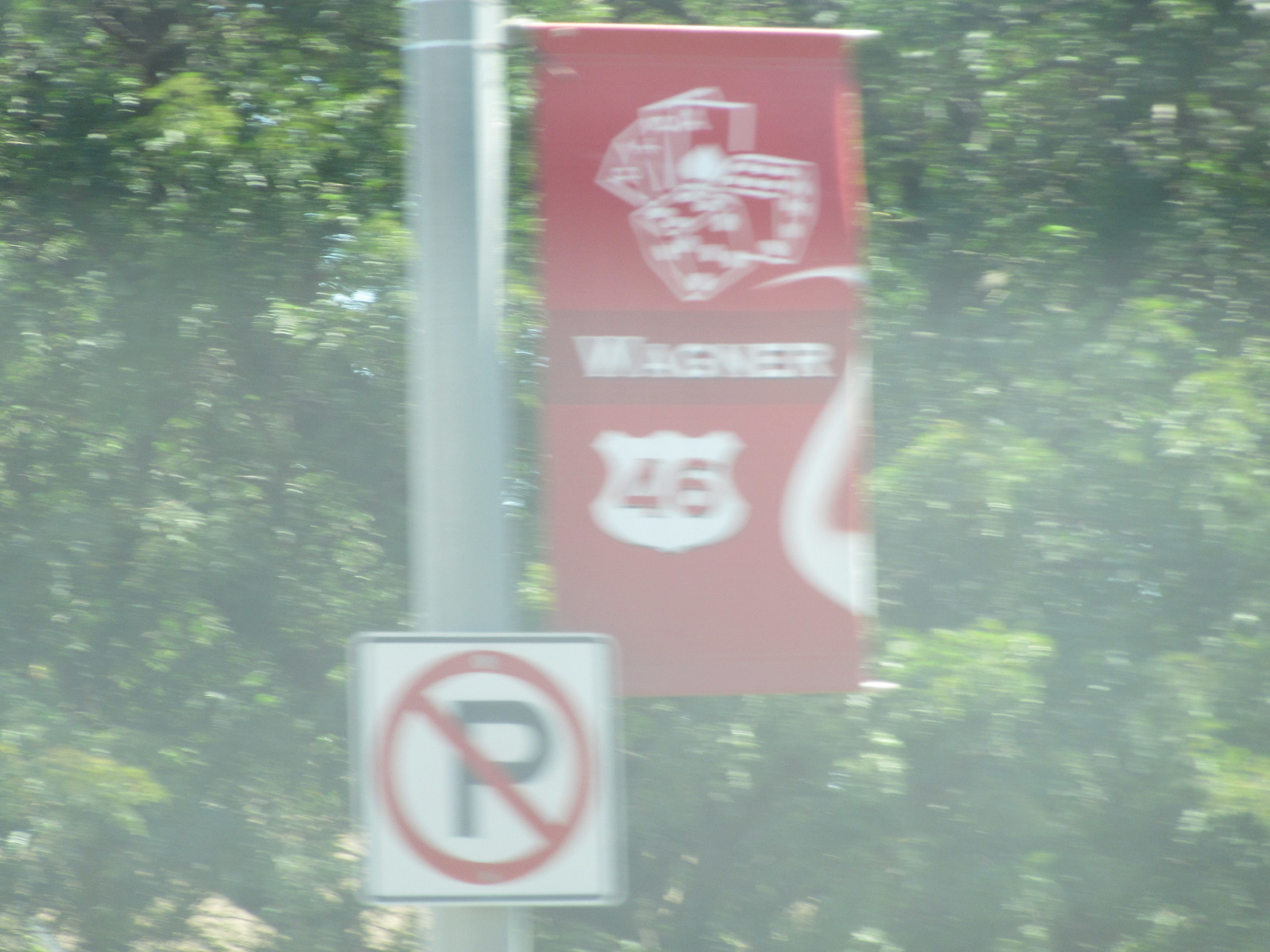This photograph features a vertical rectangular flag prominently displayed on the side of a silver light pole. The flag, which is red with white detailing, shows the text "Wagner 46” along with the interstate highway logo for Interstate 46. Additionally, it includes illustrations of dice and playing cards at the top, rendered in white. The flag is mounted on the light pole via a horizontal attachment. Below the flag, the light pole is adorned with a white square sign bordered in black, featuring a no parking symbol. This symbol is a red circle with a line through it overlaying a black letter 'P'.